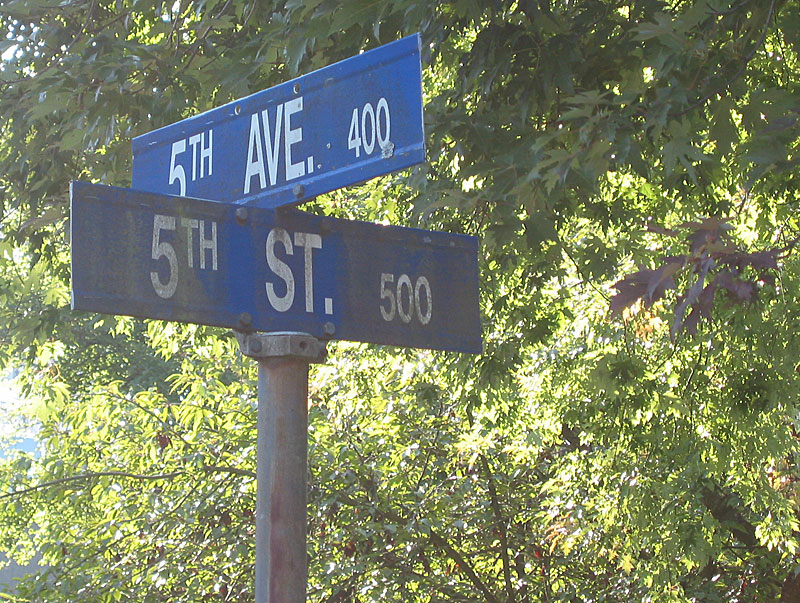A street sign marks the intersection of 5th Avenue and 5th Street, with the signage colored a mid-blue and featuring white lettering. The 5th Avenue sign reads "5th Avenue 400" and appears to be in good condition, while the 5th Street sign shows noticeable wear and tear. Both signs are affixed to a silver metal pole that displays signs of rust and has a red streak running up its length. In the background, a variety of trees, possibly maple trees, are visible. The majority of the trees have green leaves, but a notable exception is a branch halfway up on the right-hand side that boasts vibrant red leaves, contrasting beautifully with the surrounding greenery.